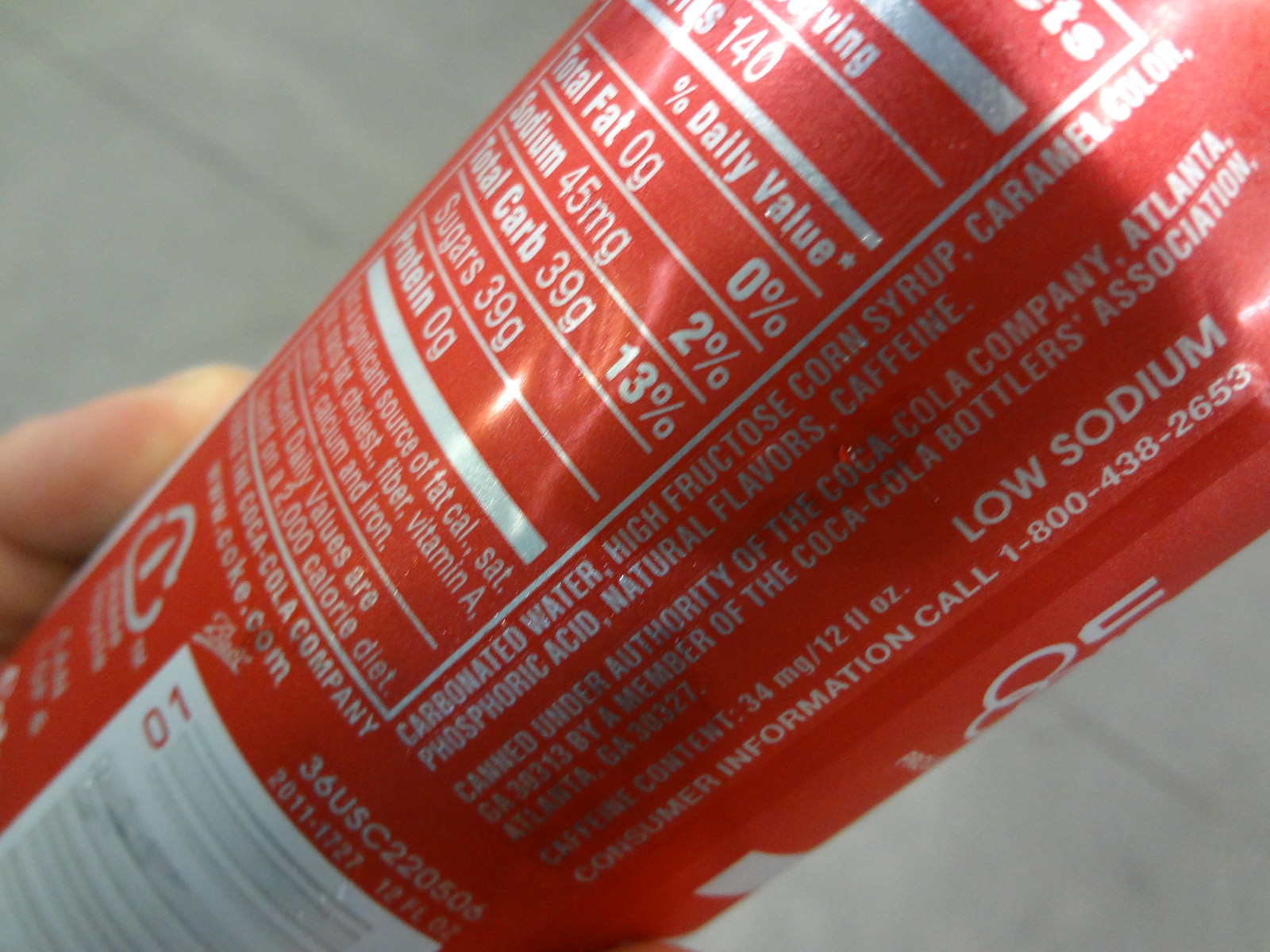The image depicts a red canned beverage, predominantly featuring silver or chrome-colored text, suggesting it might be a Coca-Cola product. The can is held diagonally by someone, with visible fingers at the bottom. The side of the can displays a list of ingredients, including carbonated water, high fructose corn syrup, caramel color, phosphoric acid, natural flavors, and caffeine. Below these, it mentions being canned under the authority of the Coca-Cola Company, with low sodium content. Additional details include a barcode at the bottom left, a nutrition facts label on the upper left, and a note to call 1-800-438-2653 for consumer information. The can's contents, such as 140 calories and amounts of fat, sodium, carbs, sugar, and protein, are partially visible. The background is a blurry, gray, possibly tiled surface. At the very bottom, a recycling symbol urges consumers to recycle the can.